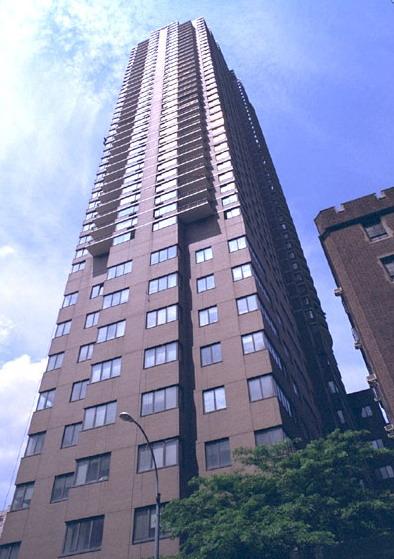This color photograph captures an expansive view of a modern high-rise skyscraper, standing at an impressive height that likely spans 40 to 60 stories. The structure largely comprises blue rectangular windows that dominate the facade, especially in the lower section. As the building extends upwards, the windows become larger and more reflective, capturing the sky’s light and creating a shimmering effect. Balconies punctuate both the left and right sides of the upper stories, gradually leading up to the building’s peak.

Nestled next to this towering skyscraper is a smaller, older brick building, providing an interesting contrast in architectural styles. Viewed from a ground-level perspective angled upwards, the image also encompasses elements of the surrounding environment: a curved street light and a leafy tree add a touch of greenery in the foreground. The sky is a brilliant blue, adorned with a couple of clouds and bathed in sunlight, particularly noticeable in the top left corner of the frame. The overall scene has a slightly faded quality, reminiscent of photographs from the 1980s.